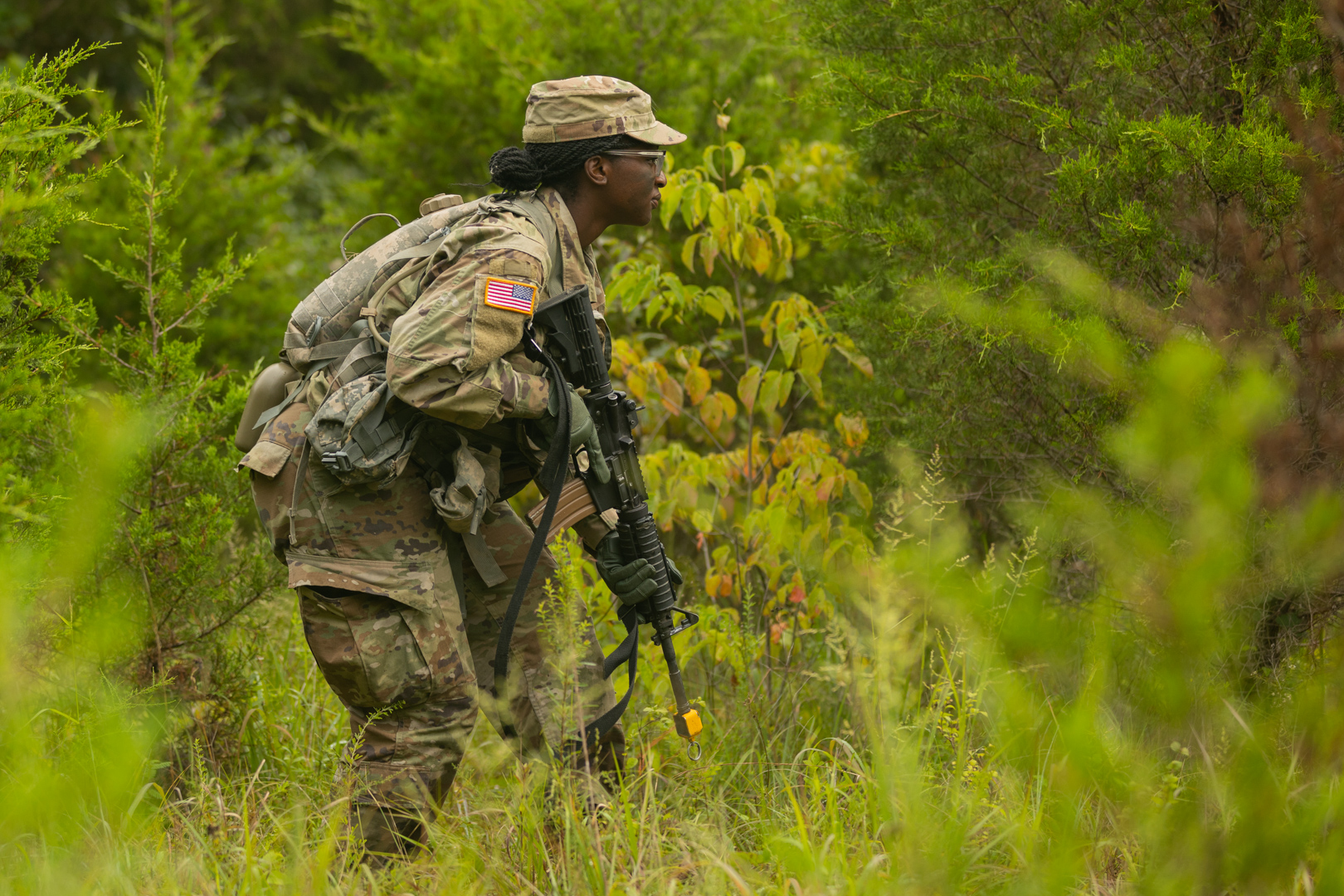In this vibrant outdoor daytime image, an African-American woman U.S. soldier is prominently featured. She is wearing a standard-issue green camouflage uniform with an American flag patch on her sleeve. Her uniform is complemented by a camouflage cap and prescription glasses. Her long braided hair is tied back neatly into a bun.

She is carrying a black rifle with a yellowish tip, the rifle pointing downward as she faces to the right. Her uniform is equipped with various essential gear, including a backpack and a water canteen, with her pockets appearing full of supplies. The background features a dense forest with a mix of evergreen and deciduous trees, predominantly showcasing healthy green foliage, though there are some yellow and orange leaves visible. Tall grasses, green with a few brown stalks, cover the ground, adding to the lush, heavily forested setting. In the foreground, a few yellowish leaves are visible, contrasting against the vibrant greenery surrounding her.